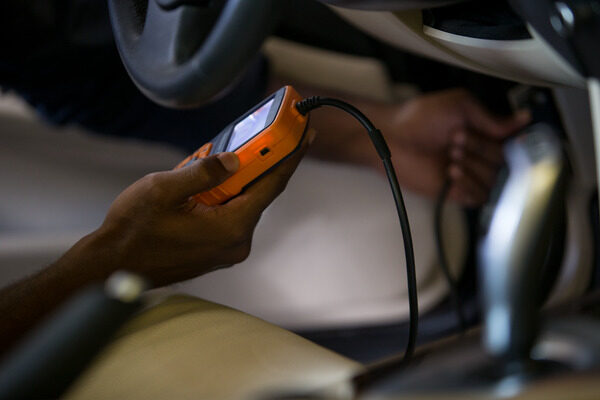In this dimly lit image taken inside a car, we see a person using a diagnostic code reader device to troubleshoot an issue. The device, bright orange in color with a small, lit screen at the top, is held in one of the person's hands. This hand is only partially visible. A thick black wire extends from the top of the device, connecting it to the car's diagnostic port. The person's other hand appears to be attaching the device to the car. On the right side of the image, the blurry outline of a gearstick is barely visible, while a part of the steering wheel and handbrake can be seen in the left and bottom left corners, respectively. The overall background features a mix of white, brown, black, and gray hues, contributing to a generally dark and indistinct atmosphere.